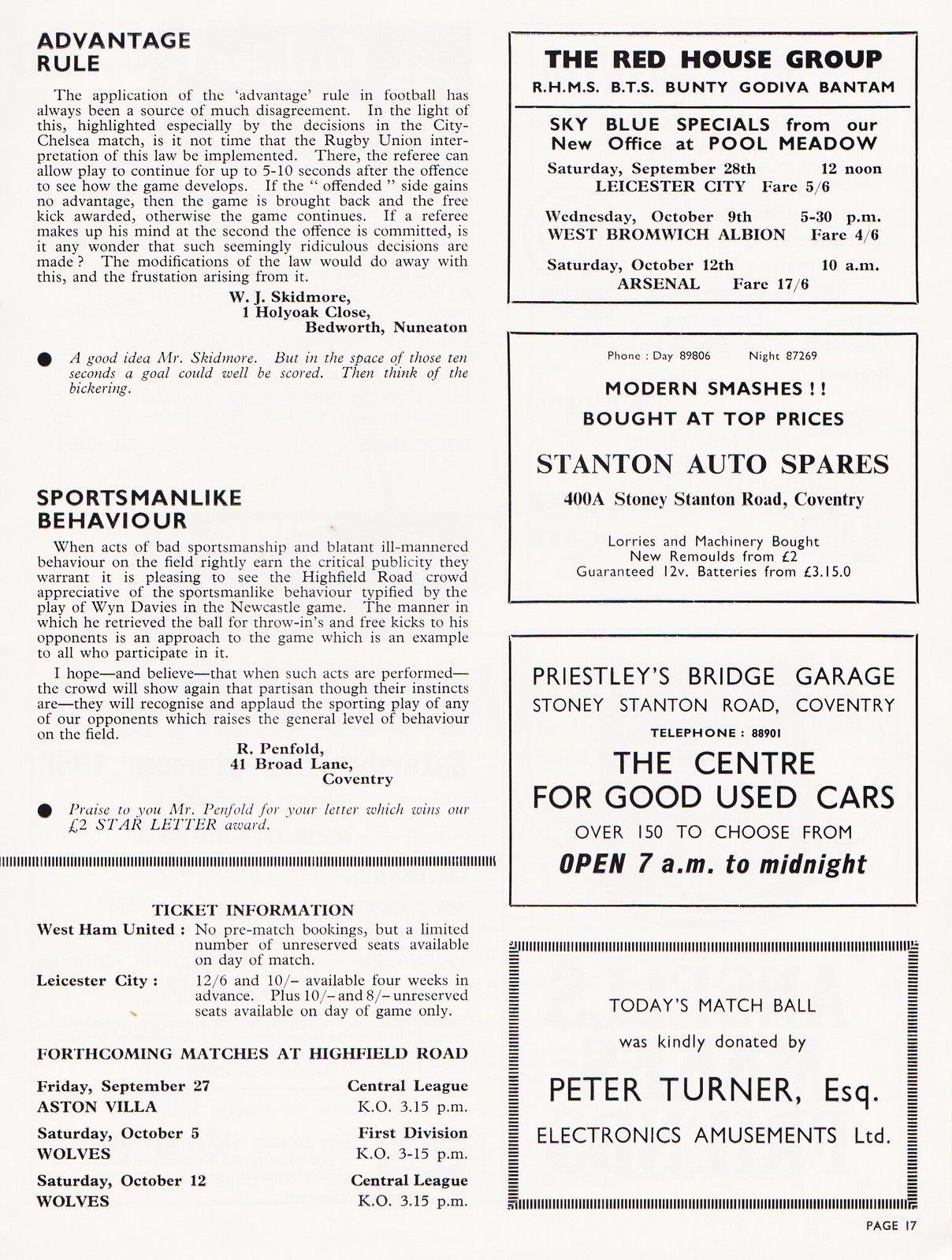This image appears to be a page from a magazine or sports program with a predominantly white background. The left-hand side features two paragraphs of text, each with its own title. The first paragraph is titled "Advantage Rule" and discusses the contentious application of this rule in football (soccer). It includes a bullet point that adds, "A Good Idea, Mr. Skidmore. But in the space of those 10 seconds, a goal could well be scored. Then think of the bickering." The second paragraph, titled "Sportsmanlike Behavior," includes a note praising Mr. Penfold, whose letter won a two-star letter award, and features the bullet point, "Praise to you, Mr. Penfold, for your letter, which wins our two-star letter award."

Below these paragraphs, there is information about ticket sales for matches featuring West Ham United and Leicester City, along with details about forthcoming matches at Highfield Road, including times and league divisions. On the right-hand side, there are four vertically aligned black rectangles with various advertisements. The first rectangle promotes "The Red House Group," the second one offers "Modern Smashes Bought at Top Prices," the third advertises "Priestley's Bridge Garage, Stony Stanton Road, Coventry," and the fourth notes that "Today's Match Ball was kindly donated by Peter Turner."